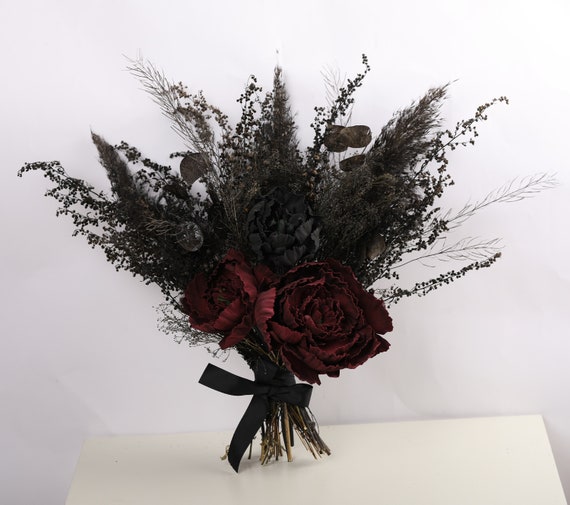The image features a dried flower arrangement resting on a white tabletop against a white wall with light gray shadows. The bouquet is composed predominantly of very dark green foliage, nearly black in appearance, interspersed with different grasses, including eucalyptus and pampas grass. The arrangement is tied together with a black ribbon into a neat bundle that stands upright without support. At the forefront of the bouquet are two large, deep crimson flowers, likely roses, which serve as the focal point. The greenery fans out in a wide V behind these prominent flowers, creating a balanced and structured composition. The photorealistic detail captures the contrast between the dark, moody colors of the bouquet and the stark, minimalistic background.